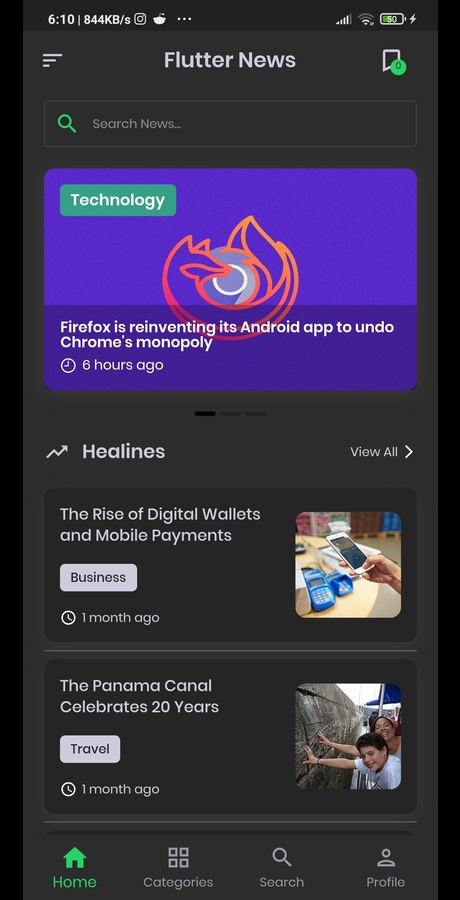A mobile phone screen displays a web page from "The Shape" featuring "Flutter News" at the top. The screen's main highlight is a large blue rectangle with a smaller green strip labeled "Technology" in white text. Within this blue section, it announces, "Firefox is reinventing its Android app to undo Chrome's monopoly," posted six hours ago. Below this headline, there is a section titled "Headlines" featuring an article on "The rise of digital wallets and mobile payments," with a "Business" category button indicating it was posted one month ago. An accompanying small image shows a person using their mobile phone at a desk. Further down, another article titled "The Panama Canal celebrates 20 years" under "Travel" was also posted one month ago; the image depicts people on one boat reaching out to touch the side of another boat in the Panama Canal.